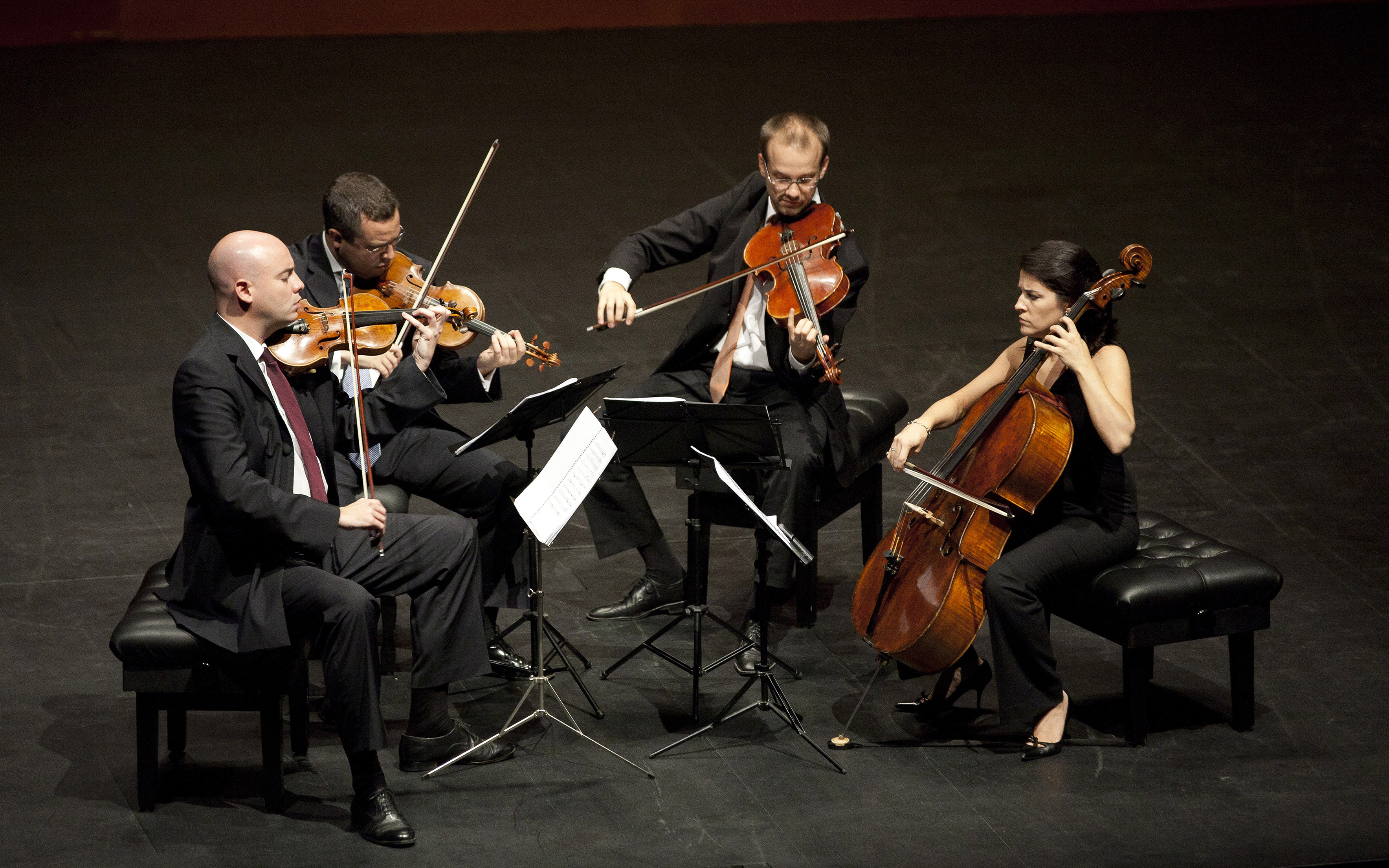In this detailed landscape photo, a symphony quartet is captured in the midst of an intimate practice session. Set against a stark black background on a dark black floor, the scene features four elegantly dressed musicians. The arrangement consists of three men and one woman. The woman, positioned at the right-hand corner, is playing a cello in a black sleeveless pantsuit. The three men, all in black suits, are playing string instruments: two violins and one viola, which is larger than the violins but smaller than the cello. Each musician is seated on a black chair, resembling a piano bench, and concentrated on their white music sheets placed on black metal music stands. The musicians form a U-shaped pattern, contributing to the sense of an intimate gathering rather than a concert, as there's no audience visible. The overall aesthetic is one of formal elegance and focused practice.